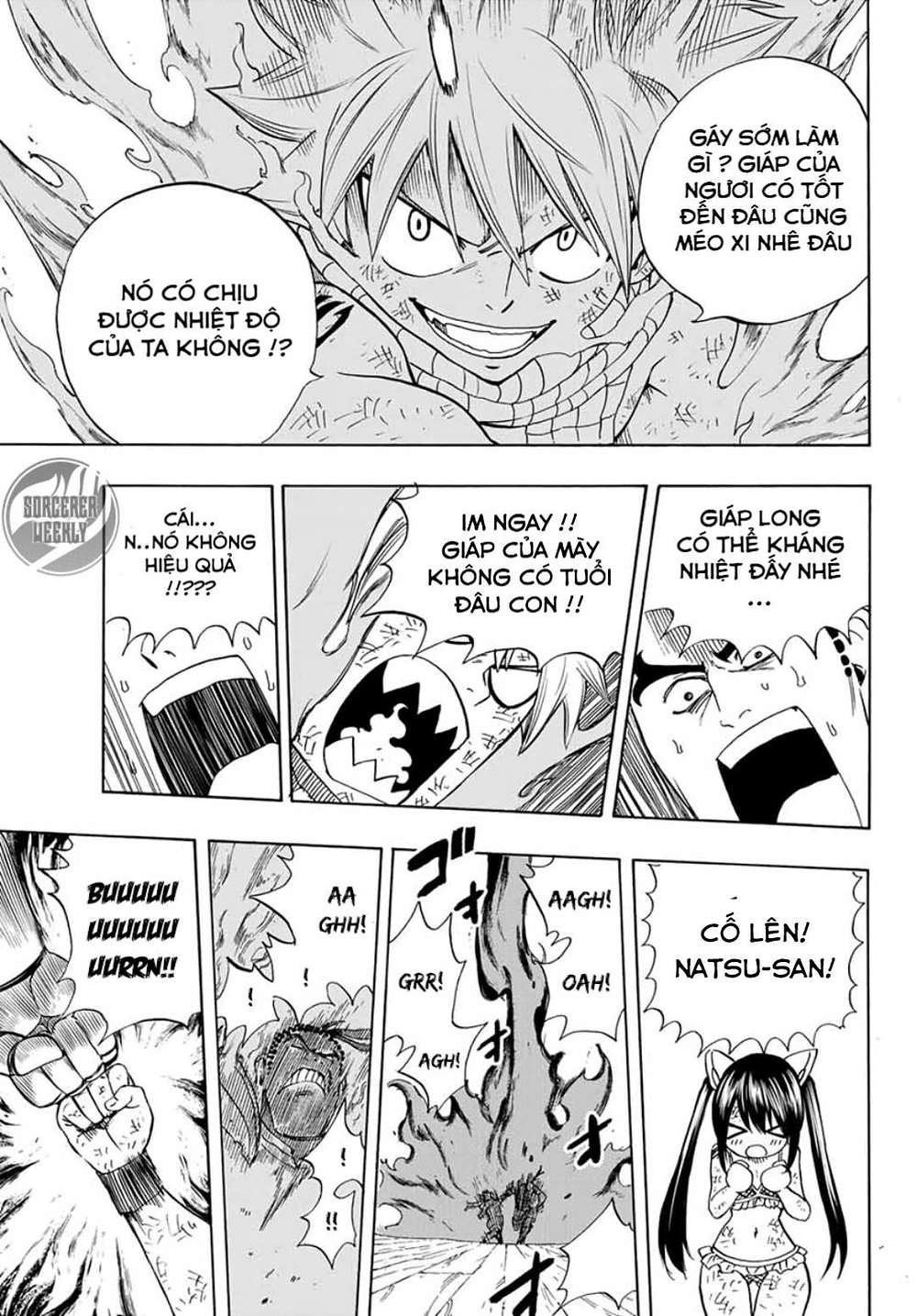This black and white comic book page is laid out in a multi-paneled format with distinct sections. At the top, there's a close-up of a gray character with spiked-down hair, wide eyes, and an open mouth, giving him a mean expression. He has speech bubbles on either side filled with text in a foreign language. Below this top panel, in the center section, there are three smaller squares. The first square contains black text at the top ending with two exclamation marks and question marks, and features an indistinguishable item with black lines and ripples above it. The next panel to the right shows a character with a wide-open mouth, sharp jagged teeth, a white flame inside their mouth, and a heavily scarred face. Adjacent to this is another character with sweat down their cheeks, black eyebrows, and a flat top row of teeth. 

The bottom section consists of four additional panels. The first displays two fists coming together with black text above ending in three exclamation marks. The next panel shows a character with a contorted face, black streaks, teeth visible through an open mouth, and expressions of pain symbolized by "ah" and "grr" with exclamation marks. To its right, a bursting flame takes center stage surrounded by "grr" and "ah" text. The final panel on the bottom right depicts a young girl with cat ears in a skimpy outfit, showing her stomach and hips, her hands together under her chin, eyes shaped like triangles, and a circular mouth. She is covered in cuts and scrapes and has thought text above ending in two exclamation marks. The various panels are well spaced, arranged in a window pane style, and contain speech bubbles in a foreign language, highlighting different shades of black, white, and gray.